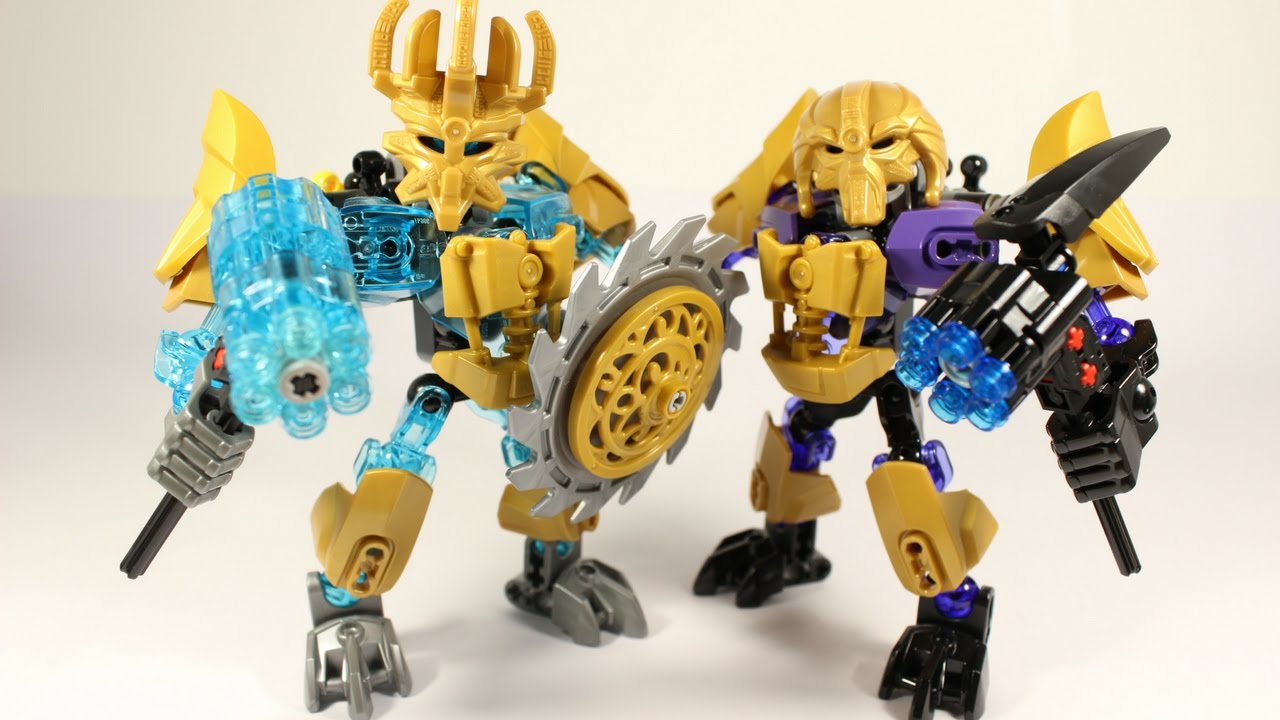The image showcases two intricately detailed Lego figures, both resembling warriors and wearing masks. The figure on the left dons a golden mask with five prongs extending upwards, creating a crown-like appearance. It wields a weapon in its right hand made of blue, clear Lego pieces, resembling the chamber of a revolver with a black staff attached. In its left hand, it holds a circular shield composed of a large silver saw blade with a golden decorative circle in front. Its legs and shoulders feature golden armor, and the lower legs and body incorporate the same blue plastic as the weapon. Silver feet complete its look.

The figure on the right mirrors the warrior aesthetic but has unique accents. It wears a mask with two downward-facing horns giving it a distinct, Predator-like appearance. This figure features purple plastic elements around its shoulders and legs, contrasting with the golden armor on its knees, chest, and shoulders. The left hand grips a weapon similar to the first figure's but made of black Lego pieces. Its feet are black, and its hands, also black, enhance the dark theme. Both figures exude a formidable presence with their heavily armed and armored designs.